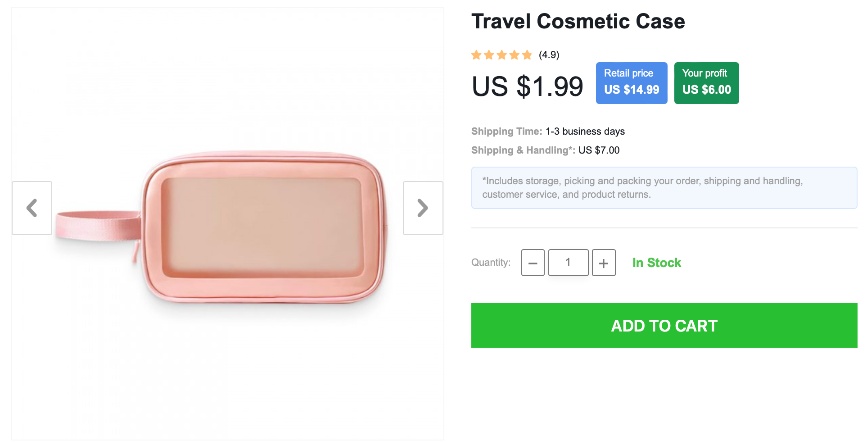This image is a cropped screenshot from a webpage displaying a travel cosmetic case for sale. The background is white, allowing the product details to be clearly visible. The main section showcases a detailed image of the pink rectangular case, which features a pink strap and a see-through front section. Flanking this image are outward-facing arrows, suggesting it’s part of an interactive gallery.

To the right of the product image, a detailed description is provided. The product title "Travel Cosmetic Case" is prominently displayed in bold black text. It boasts an impressive star rating of 4.9 out of 5. The cosmetic case is priced attractively at $1.99, marked down from a retail price of $14.99, which is highlighted in a blue box. Additionally, the potential profit margin is displayed in a green box as $6.

The shipping details indicate a quick delivery time of 1-3 business days, with an associated shipping and handling fee of $7. Below these details, there is a quantity box for customers to adjust the number of cases they wish to purchase, and an "In Stock" status is clearly noted in green text.

At the bottom of the right-hand section, a large green rectangle button invites users to add the product to their cart, making the purchasing process straightforward and user-friendly.